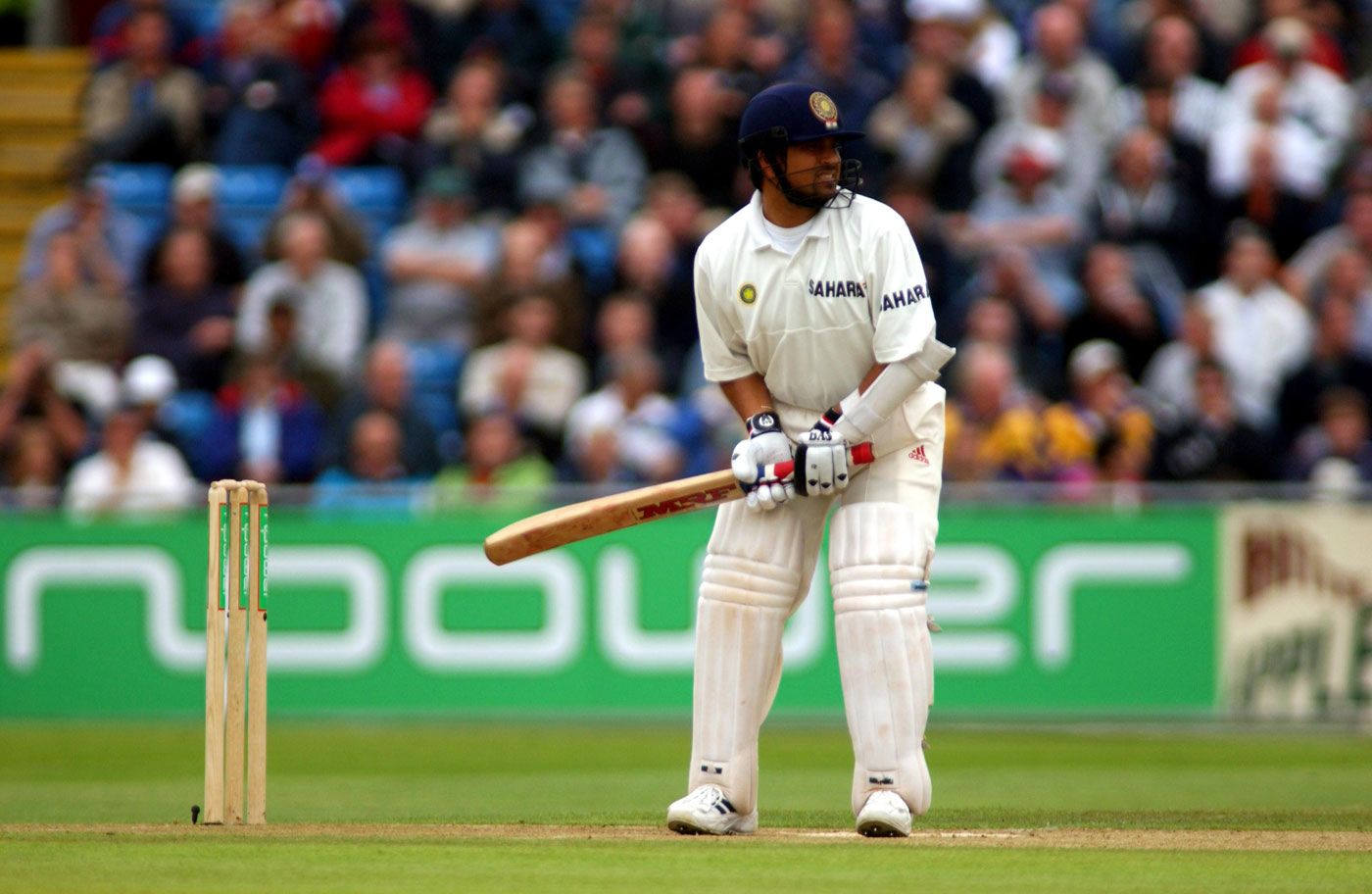In this image, we see a cricket player poised for action. The athlete is dressed in an all-white uniform complemented by thick, white gloves and padded leg guards. His helmet, which includes a protective face guard, is blue with a yellow logo. He grips a cricket bat that features red writing, and his white Adidas shoes are visible as he stands on a mixture of dirt and grass. His shirt and shoulder both prominently display the word "Sahara." The background reveals a blurred crowd seated in the stands, along with a green advertising banner, likely a sponsor logo. Most colors in the image include shades of white, brown, and green, with occasional yellow from the audience’s clothing. The scene captures the intense, focused moment just before the batter makes his play.